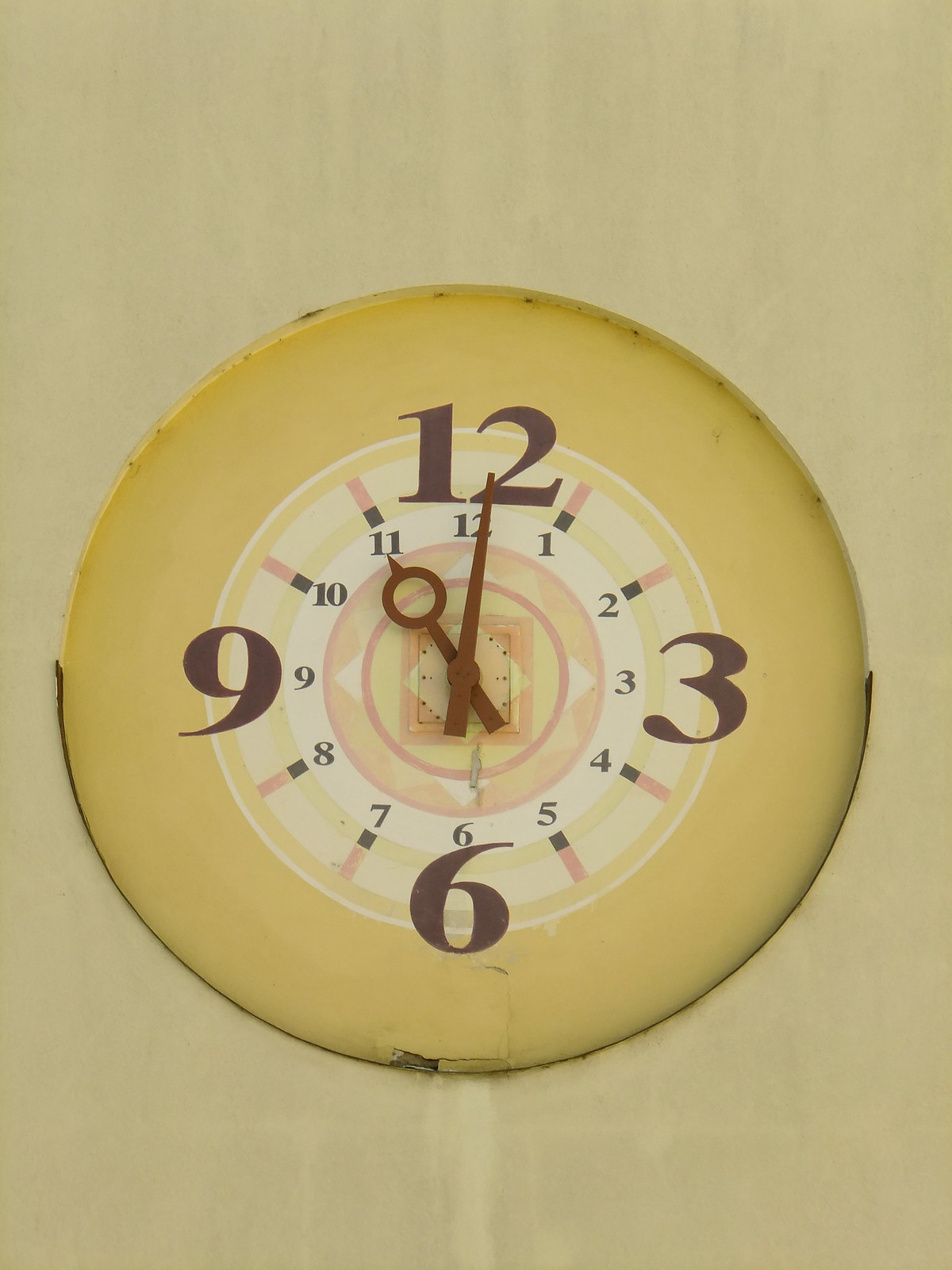This photograph features a vintage clock that exudes an old-world charm with its faded appearance and yellowed plastic casing, indicative of years gone by. The clock, rendered in an almost art deco style, showcases wide, stylized numerals that add a touch of sophistication. The larger numerals—12, 3, 6, and 9—prominently mark the quarter hours, while smaller numerals representing all12 hours are centrally positioned, providing a complete time-telling framework. Salmon-colored accents highlight the numerals, adding a subtle pop of color. The clock's hands are crafted from wood, further enhancing its nostalgic, artisanal feel. Notably, there are visible cracks in the plastic near the bottom, specifically below the numeral 6, adding to the clock's vintage character and storied history.